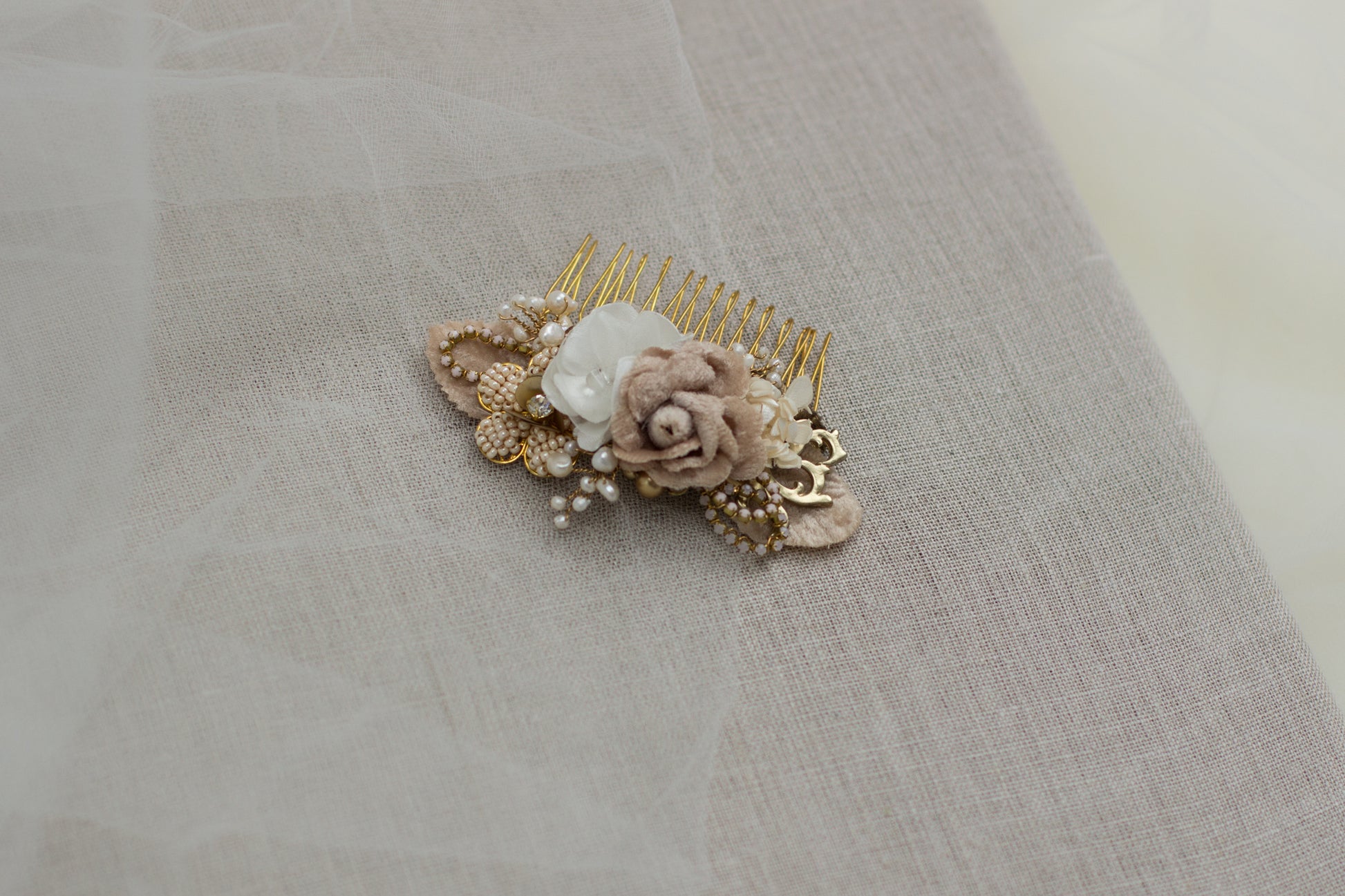In this photo, a vintage hair clip showcasing intricate craftsmanship is displayed on a delicate fabric backdrop, possibly a piece of brown linen or a woman's blouse. The clip prominently features a vibrant arrangement of elements, including a large central rose-like flower made of pinkish fabric and a juxtaposed white one that might be a feather or a similar floral accent. To the side, clusters of small pearl-like beads resemble bunches of grapes, adding a touch of elegance and detail. These beads are nestled between what appear to be the bases of leaves, subtly intertwined in the design. 

The hair clip is further adorned with golden twisty metal pieces that extend from the top, imparting a luxurious touch. Below, additional feather-like components extend diagonally, blending seamlessly with the overall motif. There are also several brass clippings and silver-colored metal pieces interwoven, enhancing its intricate appeal. The muted tones of browns, whites, and taupes lend an heirloom quality to the piece, suggesting it might be a cherished accessory passed down through generations, possibly as a "something old" for a bride. The clip's sophisticated design and detailed elements make it a striking and timeless piece of jewelry.